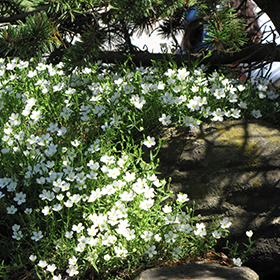This photograph captures a lush, green, wooded area on a sunlit day. The scene is taken from within trees and bushes, creating a natural canopy that filters the sunlight, casting a mix of dappled light and shadows on the ground. The centerpiece of the image is a large, vibrant green bush adorned with numerous small white flowers, occupying the lower three-fourths of the frame. Beyond this bush, a partial view of a pine tree can be seen with a striking royal blue bird perched on one of its branches. The bird faces away, adding a charming element to the serene landscape. The ground and surrounding foliage are gently illuminated by the sun, enhancing the picturesque beauty of this likely backyard setting.